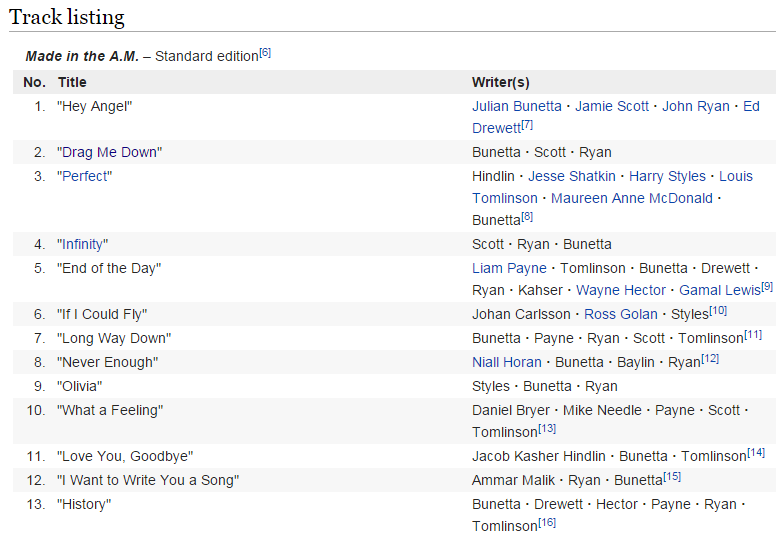A screenshot of a Wikipedia tracklisting page is shown, specifically from the desktop version of the website. The background is white, and the text is organized in a clean and structured manner. At the top left corner, the heading reads "Tracklisting," followed by a horizontal line separating it from the content below. The list comprises 13 items under the heading "Made in the A.M. (Standard Edition)."

Each track is numbered from 1 to 13, with columns labeled "Number," "Title," and "Writers." The information for each song is detailed as follows:

1. **Hey Angel** - Written by: Julian Bunetta, Jamie Scott, John Ryan, Ed Drewett (with a hyperlink denoted as [7])
2. **Drag Me Down** - Written by: Bunetta, Scott, Ryan (with a hyperlink [8])
3. **Perfect** - Written by: Jesse Shatkin, Harry Styles, Louis Tomlinson, Maureen McDonald, Bunetta (with a hyperlink [8])
4. **Infinity** - Written by: Scott, Ryan, Bunetta 
5. **End of the Day** - Written by: Liam Payne, Tomlinson, Bunetta, Ryan, Jacob Kasher, Wayne Hector, Gamal Lewis (with a hyperlink [9])
6. **If I Could Fly** - Written by: John Carlsson, Ross Golan, Styles (with a hyperlink [10])
7. **Long Way Down** - Written by: Bunetta, Payne, Ryan, Scott, Tomlinson (with a hyperlink [11])
8. **Never Enough** - Written by: Niall Horan, Bunetta, Ryan, Tomlinson (with a hyperlink [12])
9. **Olivia** - Written by: Styles, Bunetta, Ryan (with a hyperlink [13])
10. **What A Feeling** - Written by: Daniel Bryer, Mike Needle, Payne, Scott, Tomlinson (with a hyperlink [14])
11. **Love You Goodbye** - Written by: Jacob Kasher, Bunetta, Tomlinson (with a hyperlink [15])
12. **I Want to Write You a Song** - Written by: Ammar Malik, Ryan, Bunetta (with a hyperlink [16])
13. **History** - Written by: Bunetta, Drewett, Hector, Payne, Ryan, Tomlinson (with a hyperlink [16])

This comprehensive tracklisting provides a detailed insight into the song titles and the contributing writers for each track in the album.